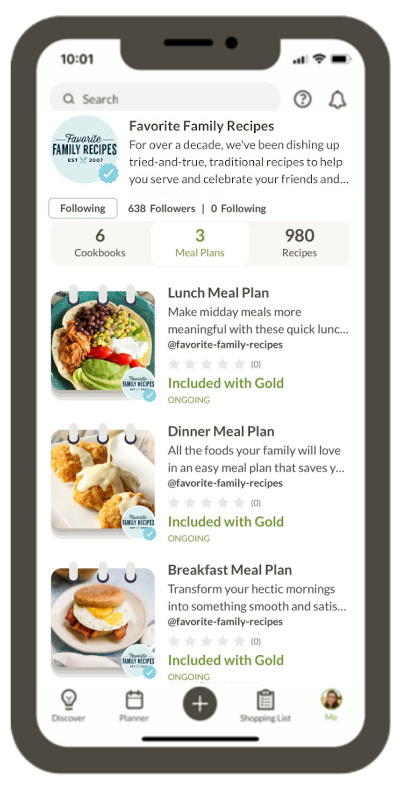The image depicts a mobile device screen displaying a family recipes app or webpage. The device has a dark gray frame. At the top left corner of the screen, the time is shown as 10:01. The upper part of the screen features a light pale off-white search bar with the word "Search" inside it, accompanied by a question mark and a bell icon to the right.

Below the search bar, there is a header that reads "Family Favorites, Family Recipes." A descriptive text beneath this header states: "For over a decade, we've been dishing up tried and true traditional recipes to help you serve and celebrate your friends and..." indicating that more text follows.

Underneath this description, there is a section indicating "638 followers, 0 following." Further down, the screen displays three smaller images of various foods with corresponding detailed descriptions on the right side of each food image. These smaller images and their descriptions give an impression of a diverse selection of recipes available within the app or webpage. The overall theme suggests a focus on traditional family recipes designed to bring people together.